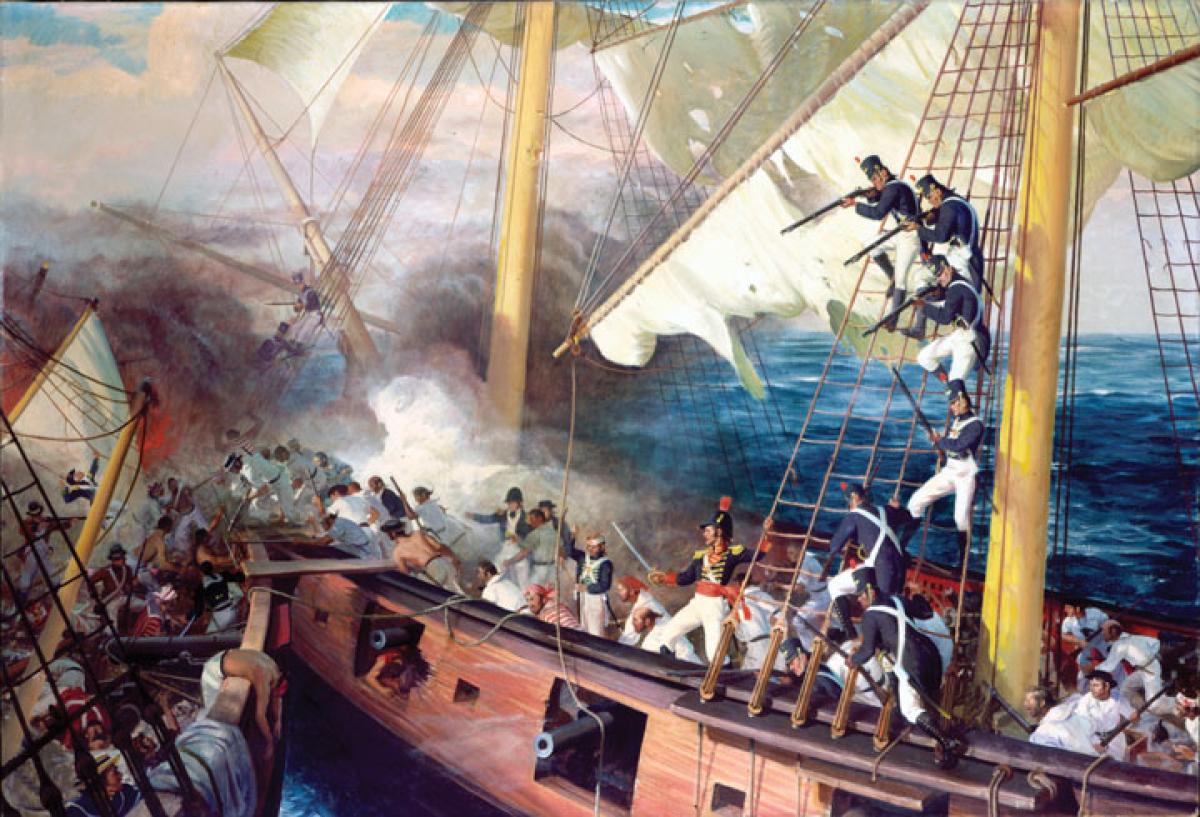This detailed painting vividly portrays an intense naval battle between two ships amidst the vast dark blue waters accented with cyan. The ships are side by side, nearly colliding, with wooden planks bridging their decks for boarding. On the left, the ship appears to have taken severe damage, with a tipped mast devoid of its flag and a fallen mast with a white flag. A thick plume of black smoke emerges from its deck, suggesting a fire. Scattered around are lifeless bodies, including a man in a red vest and white pants, another shirtless man in white pants draped over the side, and several others in white shirts.

The second ship to the right is teeming with action. Its crew, clad in long-sleeve blue shirts with white stripes, white shirts, and some in distinctive red coats and white pants, are aggressively boarding the left ship. Many are climbing the large masts with two prominent white sails, with their muskets drawn and aimed downward, while one man with golden accents on his attire, likely the captain, brandishes a sword in the air, rallying his men for battle. The sky above is a cyan backdrop with thick white clouds, intensifying the drama of this historic clash. The contrasting uniforms hint at a specific naval force, possibly British or French, suggesting the painting might be inspired by an actual historical encounter.